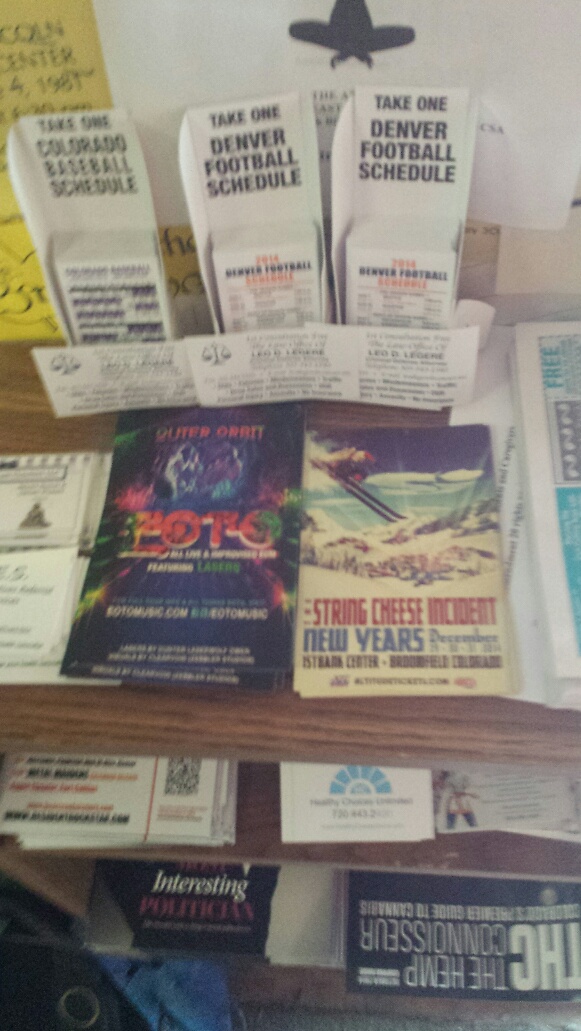The image features a crude, darker brown wooden stand, which looks like a bookshelf or a display with multiple shelves. The stand is filled with a variety of items, including flyers, posters, magazines, and loose papers. Despite the low-quality and blurry nature of the photo, some details are discernible. Prominently, there are white pamphlets with inscriptions such as "Take one: Denver football schedule," "Take one: Colorado baseball schedule," and a repeated mention of taking a Denver football schedule, including a specific reference to the 2014 Denver football. Additionally, the content on the shelves includes a poster for a music event titled "String Cheese Incident, New Year's" and another poster labeled "Outer Orbit FOTO featuring lasers." The stand also holds several magazines, including one titled "The Hemp Connoisseur: THC Magazine," and a book with the title "Interesting Politician." The overall appearance resembles that of an information stand one might find in a tourist center or rest stop, filled with a mix of regional schedules, event flyers, and reading materials.